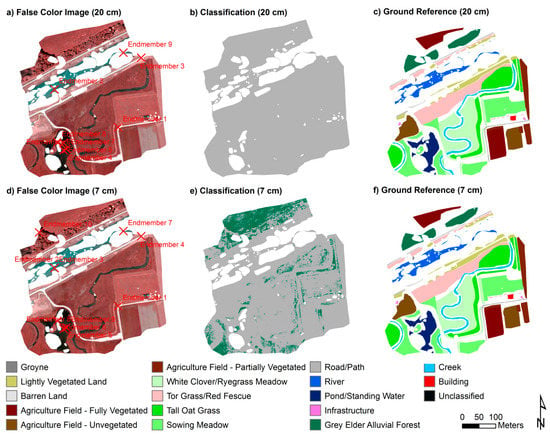The image, resembling a textbook or official document, displays six scientific depictions of a landscape segment, arranged in a 2x3 grid. Each column and row provides different visual perspectives and classifications of the landscape at varying resolutions. The left column features reddish hues labeled "False Color Image" at 20 cm and 7 cm. The center column shows gray-scale images, marked "Classification" at 20 cm and 7 cm. The right column displays multicolored maps titled "Ground Reference" at 20 cm and 7 cm. Below these images, a detailed key lists various colors corresponding to landscape features: bright green for "Tall Oak Grass," light green for "White Clover/Ryegrass Meadow," dark blue for "River," navy blue for "Pond and Standing Water," bright red for "Building," among others including "Unclassified" in black. This detailed representation aids in understanding different land use types and vegetative cover in the depicted area.